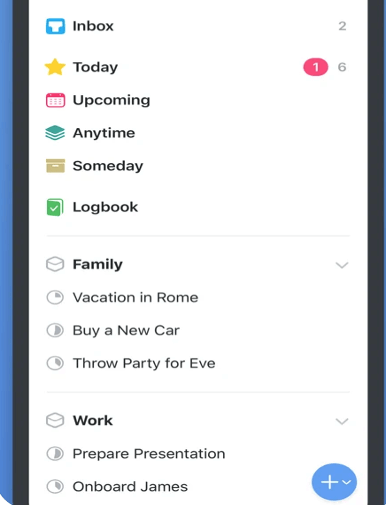This is a close-up screenshot of a mobile screen displaying a pop-up menu with parts of the display cut off on all sides. On the left edge, there's a vertical black bar adjacent to a purple bar. The primary screen area is white. At the top of the pop-up menu, the word "Inbox" is prominently displayed in black font alongside a blue square icon featuring a white "T".

Further right, in gray font, the screen reads "To" followed by "Today" beneath it. To the left of "Today" is a five-pointed yellow star icon, and to the right, there's the number "1" encircled in red, followed by the number "6" in gray. Below this, the screen displays "Upcoming" next to a calendar icon, then "Anytime" next to an icon depicting three stacked pieces of paper, and "Someday" next to a filing cabinet icon. Beneath this section, it says "Logbook" with a notebook icon beside it.

A horizontal gray line divides the "Logbook" section from the subsequent list items. Below the line, the categories and items listed are "Family" which includes "Vacation in Rome", "Buy a new car", and "Throw a party for Eve". Another gray line separates these categories from the "Work" section, which includes "Prepare presentation" and "Onboard James".